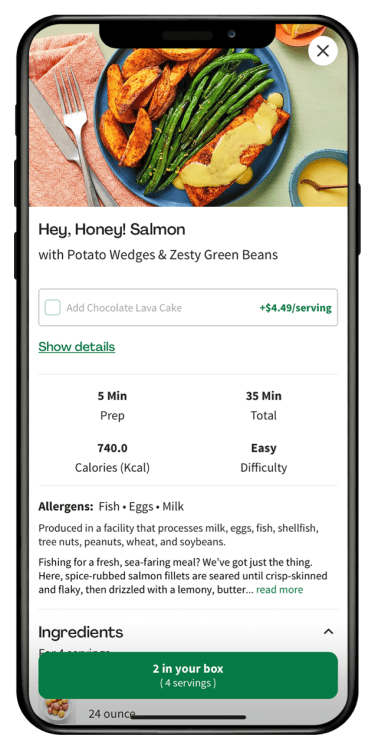The image appears to be a mouthwatering advertisement or promotional screen for a salmon dish. It is displayed on a black-outlined phone, which has three black buttons on the left side, one black button on the right, and a black oval at the top, possibly for a front camera.

At the upper portion of the screen, there is an appetizing picture of a meal consisting of:
- A folded orange or light reddish handkerchief on the left side, adorned with a neatly placed fork and knife.
- Positioned centrally is a blue round plate filled with delicious food. The plate contains:
  - Salmon covered with a yellow sauce.
  - Crisp green beans.
  - Golden potato wedges.
- At the bottom right, there's a small sauce bowl with a round spoon in it, containing the same yellow sauce.

Below this image, the background transitions to white with black text. The caption reads:
"Hey honey, salmon with potato wedges and zesty green beans."

Encapsulated within a gray-bordered white rectangle, additional details are offered:
- "Add chocolate lava cake" in bold, with a green plus symbol indicating an additional cost of $4.49 per serving.
- Below is a green link reading "Show details."

A thin gray line demarcates this section from the nutritional information:
- "5 MIN prep, 740.0 calories (KCAL)"
- "35 minutes total"
- "Easy difficulty"

A second thin gray line follows, leading into allergen warnings:
- "Allergens: fish, eggs, milk"
- "Produced in a facility that processes milk, eggs, fish, shellfish, tree nuts, peanuts, and soybeans."

Below this, an enticing description reads:
"Fishing for a fresh seafood meal? We've got just the thing. Here, spice-rubbed salmon fillets are seared into crisp skin and flaky flesh, drizzled with honey-lemon butter."

The text continues with a green "Read more" link.

Finally, at the bottom of the screen, a green box states:
"$20 a box, 4 servings."